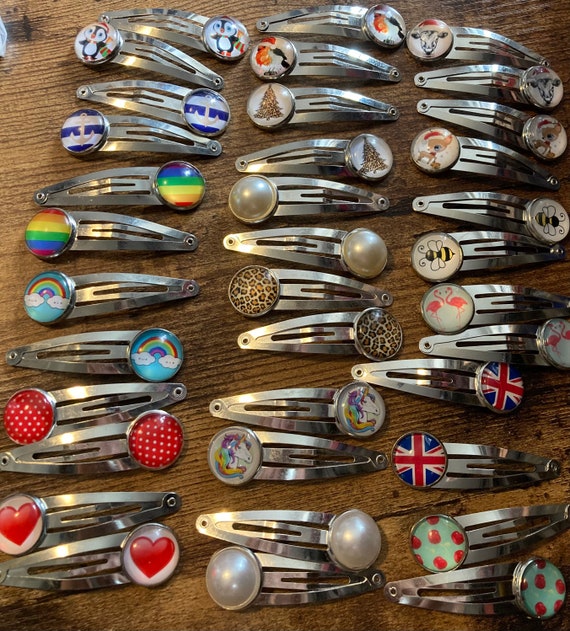The image showcases a collection of 33 silver-colored hair clip barrettes, meticulously arranged in three rows with 11 barrettes per column. Each barrette features a circular design at the end, adorned with a variety of intricate and colorful images or symbols. The designs range from penguins and cows wearing Santa hats, to hearts, a rainbow flag, the British Union Jack, Christmas trees, and strawberry textures. These distinctive barrettes are neatly displayed on what appears to be a wooden surface, likely a table or desk, and the photograph captures a directly overhead view, emphasizing the detailed craftsmanship and variety of the hairpins, suggesting that they might be collector's items.